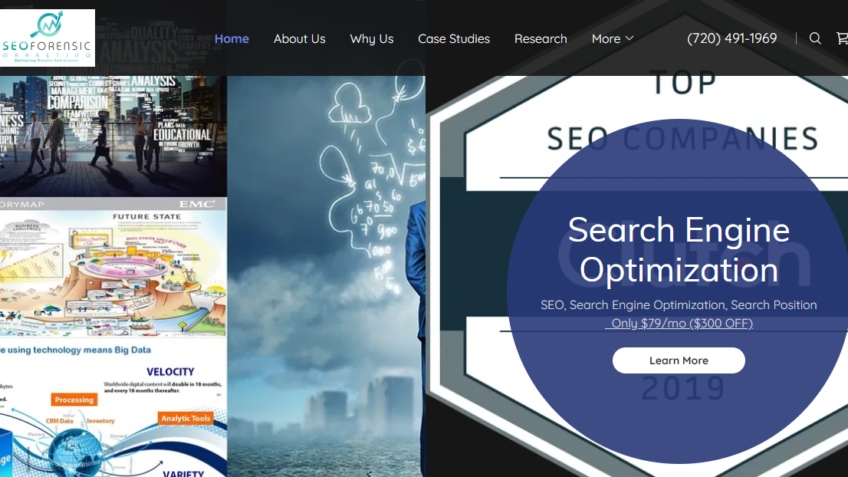A detailed caption for the image could be:

"The screenshot depicts a comprehensive SEO website titled 'SEO Forensic.' The website features a wide, desktop-oriented layout. At the top, a primary navigation toolbar lists sections: Home, About Us, Why Us, Case Studies, and Research. A prominent pop-up overlay bubble advertises a special offer for search engine optimization services, with a highlighted message stating 'Search Position, Only $79 a Month, $300 Off,' accompanied by a white pill-shaped 'Learn More' button.

The visual composition of the image is eclectic, combining various elements. On the left, there is a stock photo of a man standing by a body of water, with a bustling downtown skyline visible across the water. The right side of the image is cluttered with intricate, abstract graphics, which seem to represent complex data or metrics but are not immediately clear in meaning. The overall presentation suggests a somewhat fragmented attempt to blend professional SEO services with dynamic, illustrative content."